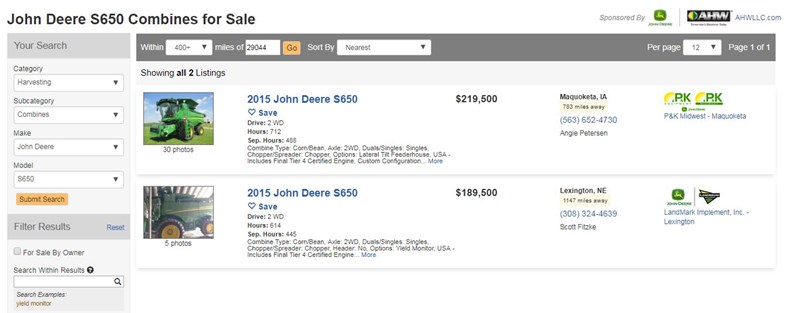This is an online marketplace dedicated to selling John Deere equipment, akin to an eBay specifically for John Deere products. The featured listing showcases two John Deere S650 combines for sale. These substantial pieces of farming machinery are priced at $219,000 and $189,000 respectively. The more expensive one appears to be in better condition. The website allows users to browse by category, such as "harvesters," and further filter by subcategories like "combines." It may offer other products as well, but the current focus is on harvesting combines. Both combines listed are from the year 2015, indicating they are used but relatively modern. This platform is particularly useful for those managing large farms and seeking specific models of John Deere machinery.